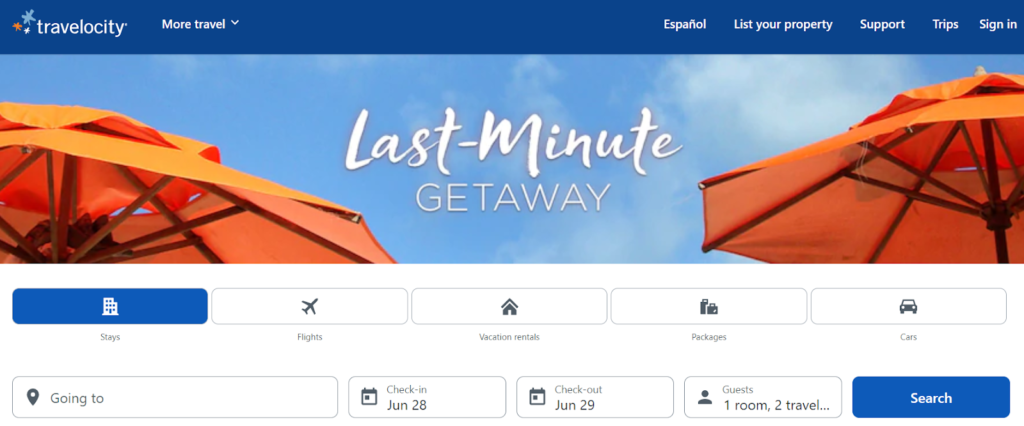The image is a screenshot of the Travelocity website's homepage. The top of the page features a blue banner with the Travelocity logo accompanied by the word "Travelocity" on the left side. Adjacent to the logo, there is a drop-down menu labeled "More Travel." Moving towards the right side of the banner, there are several options: "Español," "List Your Property," "Support," "Trips," and "Sign In," in that order.

Beneath the blue banner, the background of the homepage displays a serene image with a clear blue sky and a few scattered clouds. Flanking the image are two vibrant orange beach umbrellas. Prominently centered on this background in bold white font is the phrase "Last Minute Getaway."

Just below this text, there is a row of five buttons. The first button, highlighted in blue with a building icon, indicates the selected option. The remaining buttons, in white with gray icons, depict an airplane, a house, luggage, and a car respectively, from left to right.

Further down, a search interface is presented. It includes a "Going To" field marked with a pin icon, a "Check In" date of June 18th, a "Check Out" date of June 29th, and a "Guests" option labeled "1 room, 2 travelers." The section concludes with a prominent blue "Search" button located in the bottom right corner.